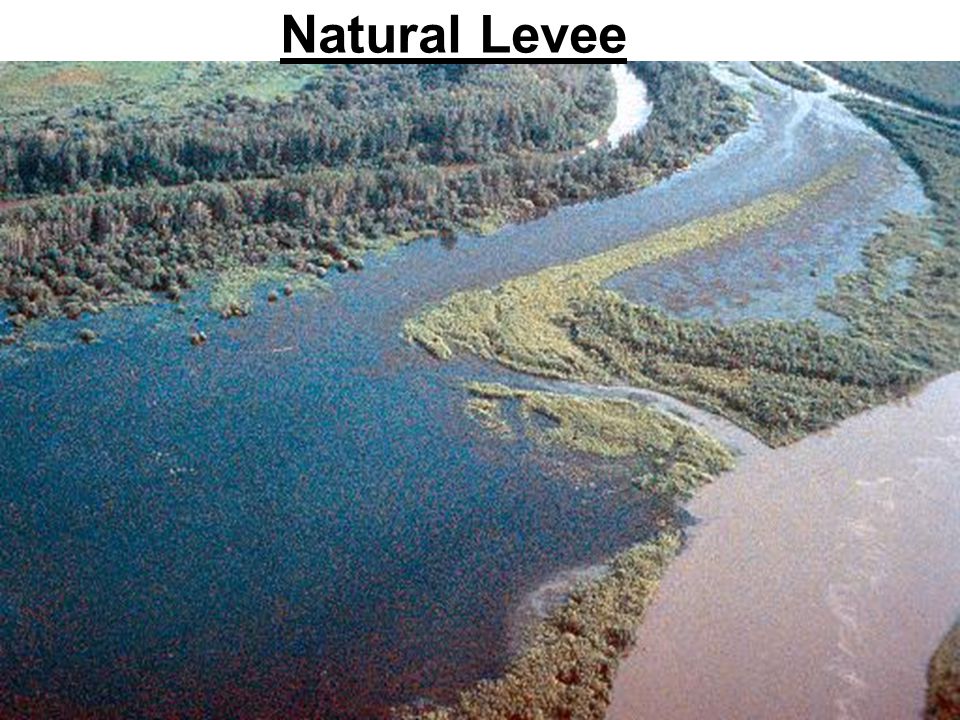The image, labeled "natural levee" in black text with an underline at the top, provides an aerial view, likely from a helicopter, of a dynamic water landscape. Dominating the center is a large swath of deep blue water, interspersed with patches of light green, suggesting vegetation or small islands within the body of water. Toward the bottom right, the water transitions into a muddy, brownish hue, indicating the mixing point with another water source. The upper left of the image is densely populated with a row of trees and green grass stretching across, while similar greenery — including shrubs and bushes — continues into the upper right-hand corner, creating a verdant frame around the water. The water bends from left to right through the scene, with additional green patches, likely vegetation, dotting its edges. The lower right of the image showcases a sandy area, adding to the textural diversity of the landscape captured.